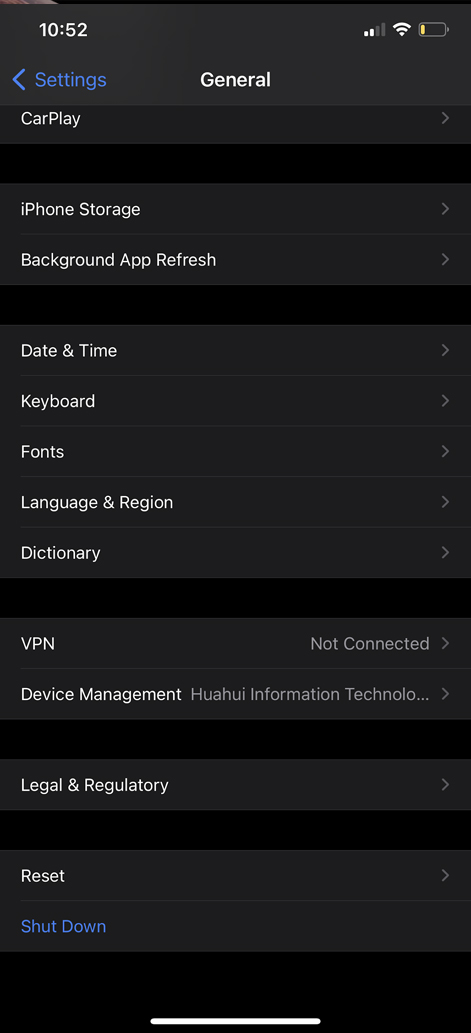A screenshot from a smartphone displaying the "Settings" menu is shown. The background is a black and gray gradient with white text. The time "10:52" is visible in the upper left corner, while the battery icon, indicating a low charge, is in the upper right corner.

In the upper part of the screen, the options "Settings" in blue and "General" in white are displayed next to one another. Below, a section lists "CarPlay," followed by a light gray area offering two choices: "iPhone Storage" and "Background App Refresh."

The following section, with a gray background, includes multiple options: "Date & Time," "Keyboard," "Fonts," "Language & Region," and "Dictionary."

Further down, there are two more settings: "VPN," which shows as "Not Connected," and "Device Management," labeled as "Huey Information Technology."

Near the bottom of the screen, another gray section reads "Legal & Regulatory." The final section features "Reset" in white and "Shut Down" in blue. The image concludes with a black border at the bottom where a small, solid white line is centered.